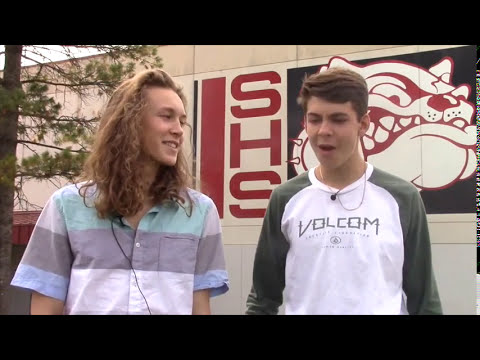The image appears to be a still from a movie or a staged scene outside of a high school campus, possibly SHS, as indicated by the letters in the background. Prominently, there's a detailed illustration of a bulldog with red highlights on its eyes, gums, and nose against a black backdrop. The setting includes an outdoor wall of the school and to the left, branches of an evergreen tree can be seen. In the foreground are two young men. The boy on the left has long brown curly hair and wears a short-sleeve button-up shirt with green, grey, blue, and white stripes. He appears to be smiling or laughing while looking at his friend. The boy on the right, wearing a long-sleeved Volcom T-shirt with white and green details, sports a microphone clipped to his collar, suggesting they might be giving an interview. Both teens exhibit a casual, yet engaging demeanor.